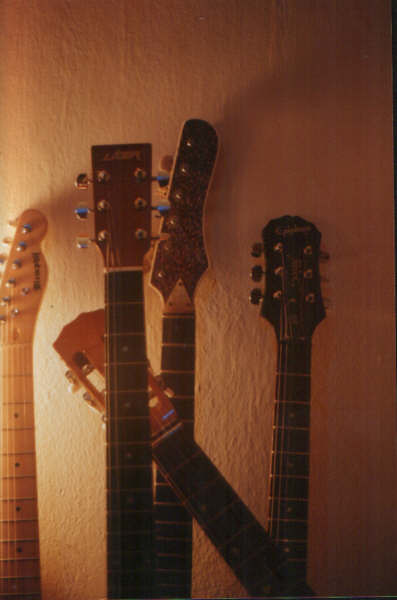This detailed photograph captures the top sections of five different guitars – likely a mix of acoustic and electric – hanging on the side of a textured, light brown wall illuminated slightly from the left. Four of the guitars stand upright, while the fifth on the far right is tilted, partially overlaid on three of the upright ones. Each guitar handle displays unique characteristics: variations in the tuners' arrangement and the shapes of their headstocks. For instance, one guitar has its tuners aligned vertically in a single row, while two others feature tuners arranged in two rows of three. The handles vary in wood tone, ranging from dark brown to light brown, and display a mix of rounded and square top shapes. The light accentuates a few of the guitar tops, highlighting their strings and distinct structural details. The arrangement and subtle lighting draw attention to the subtle differences and craftsmanship in each guitar's design.